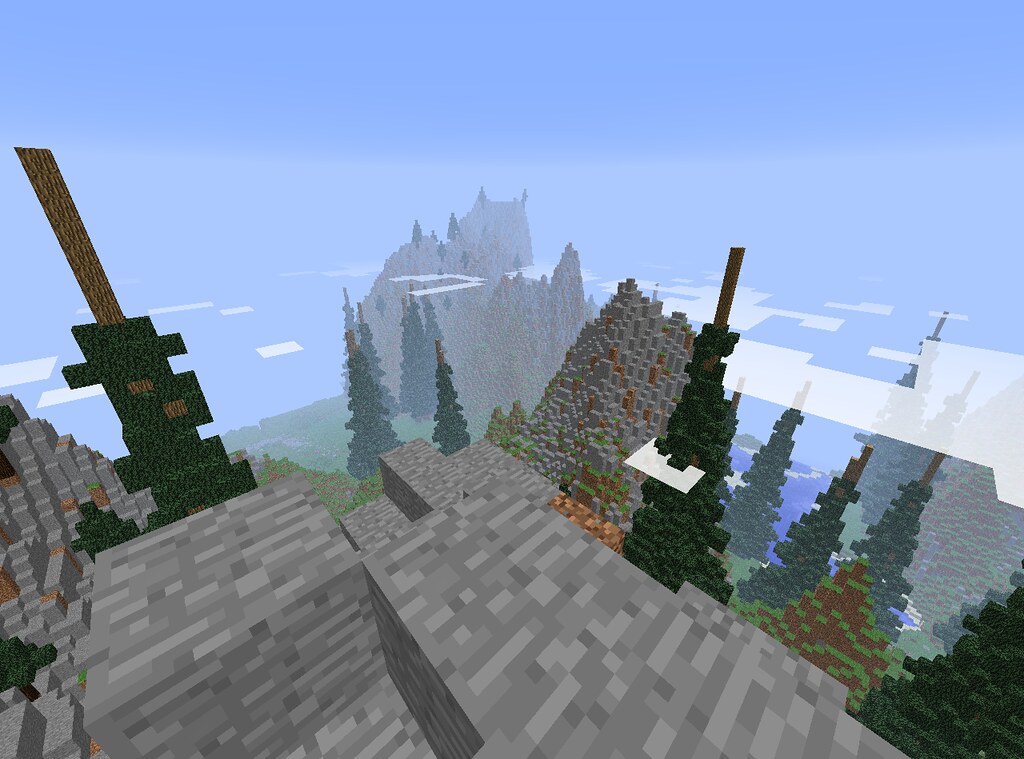This digital artwork portrays a richly detailed, three-dimensional fantasy world crafted from Lego-like shapes. The lower half of the image features a labyrinth of dark and light gray blocks, meticulously assembled into an array of geometric walls and structures. Toward the far left background, rectangular and square blocks form an intricate skyline of additional walls or buildings, enhancing the sense of depth. Diagonally aligned, pine tree-shaped structures emerge from beyond these walls on the right, adding an organic contrast to the rigid geometry. Distant, cliff-like mountains rise majestically, with small trees scattered at their base, emphasizing the vastness of the scene. The upper corners of the image are bathed in shades of blue, which could symbolize either sky or water, further immersing the viewer in this fantastical realm. The overall aesthetic is reminiscent of a carefully crafted video game environment, blending imaginative architecture with natural elements.